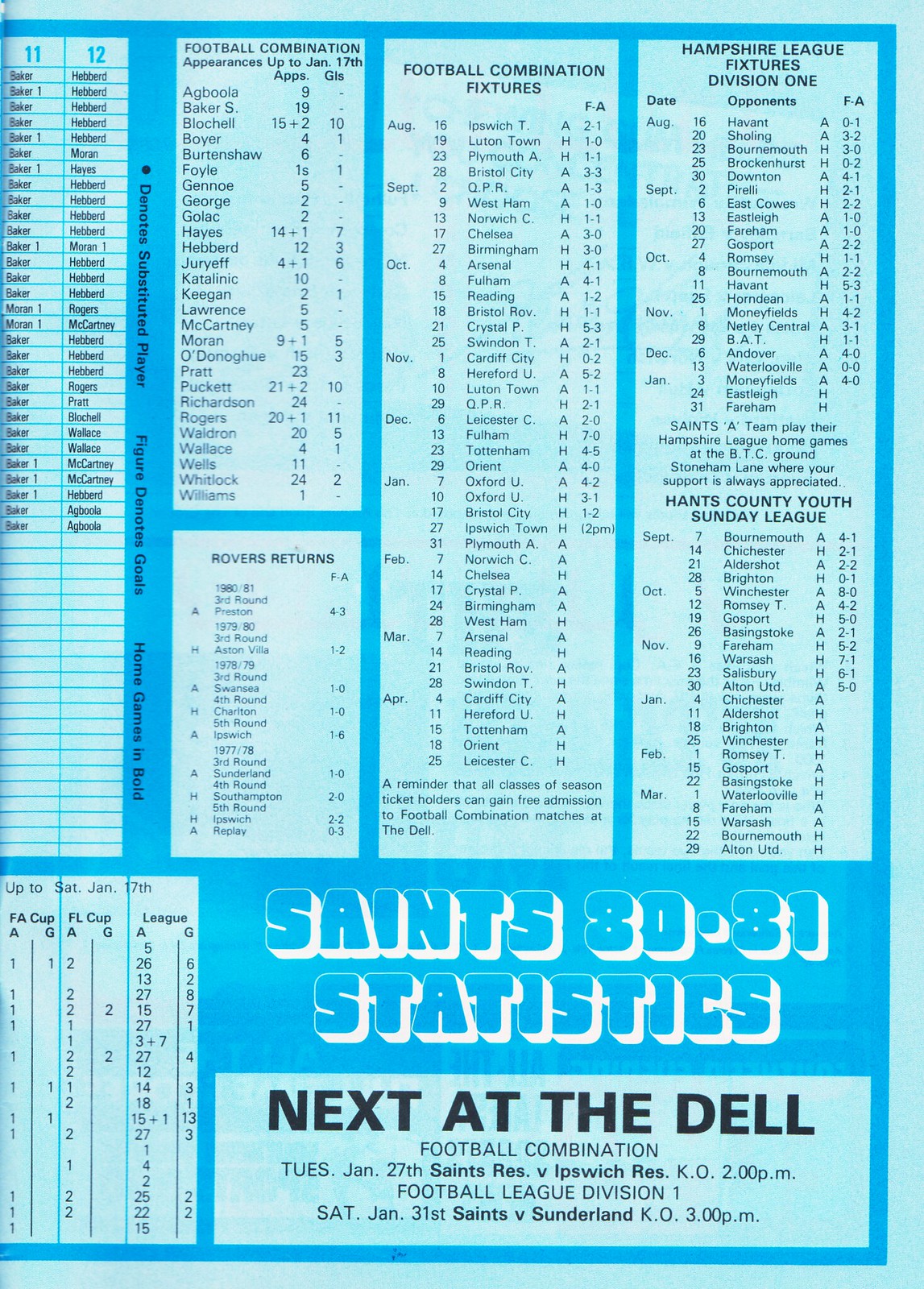The image is a text-based handout with information about a soccer event. The background is dark blue, and the image features several light blue rectangular sections with black text. At the top of the image, there are 4 to 5 rectangular sections that list various football combinations and fixtures, with columns labeled "Football Combination," "Football Combination Fixtures," and "Hampshire League Fixtures." There is another column to the left with numbers 11 and 12, and additional boxes and statistics below. On the bottom left side, there is one more rectangular section. The bottom right side of the image reads "Saints 80-81 Statistics" in 3D letters with a white outline. Below that, it states "Next at the Dell Football Combination" in larger black font, followed by smaller text listing scheduled matches: "Tuesday, January 27th, Saints vs. Ipswich Reds, Kickoff 2:00 PM" and "Football League Division 1, Saturday, January 31st, Saints vs. Sunderland, Kickoff 3:00 PM."